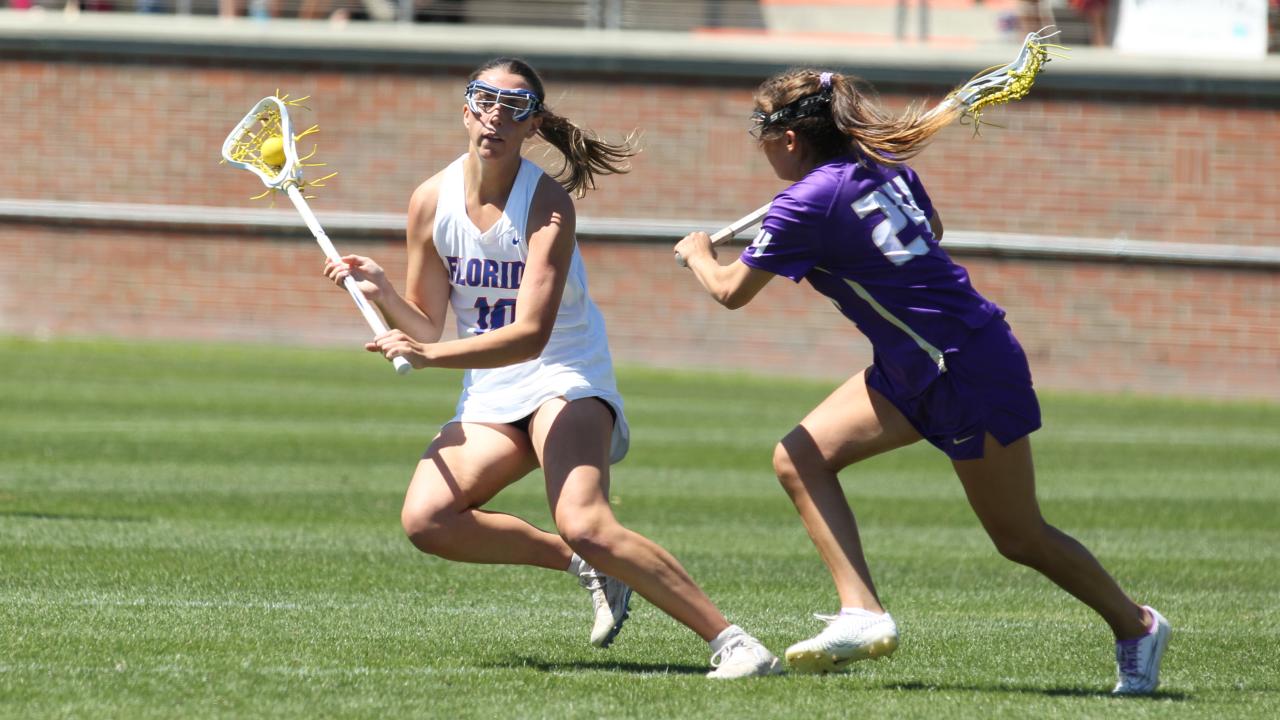This detailed color photograph captures an intense moment during a women’s lacrosse match on an artificial grass field, which features alternating lighter and more desaturated bands. At the forefront, the player on the left, with long hair tied back in a ponytail and sporting protective goggles, dons a white tank top with "Florida" emblazoned in blue text outlined in red, along with number 10. She is holding a white lacrosse stick that has a yellow basket cradling a yellow ball. The player to her right, identifiable by her purple jersey marked with the number 24 in white text, is seen from the back as she chases the ball carrier, her identical stick poised but empty. Both athletes are equipped with white sneakers fitted with cleats for traction on the turf. In the background, a brick wall with a concrete top, composed of red and gray bricks, completes the scene, adding structural context to this dynamic sporting event.